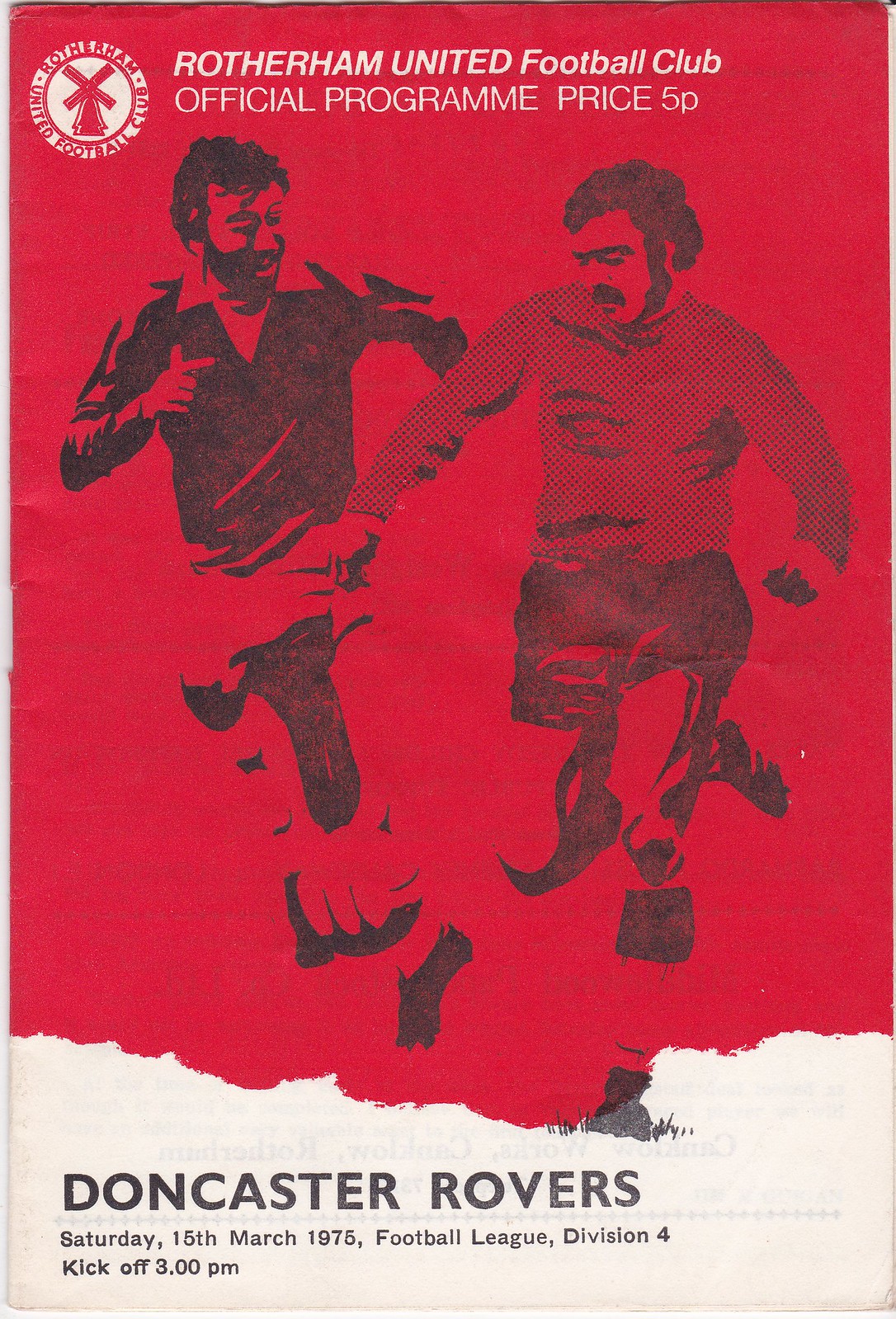The image appears to be the cover of a vintage magazine or pamphlet, presented in a 9.5 by 11-inch style typical of a book. Dominated by a striking red background, it features two silhouetted soccer players engaged in a tussle for possession of a red ball with a touch of black at its base. The player on the left is dressed in a black uniform, while the player on the right wears a slightly darker red uniform, blending seamlessly with the background. The top of the cover displays the title "Rotherham United Football Club Official Program Price 5P" in bold white letters. A logo occupies the top left corner, consisting of a white circle with a red windmill forming an 'X' pattern, beneath which is the windmill's tower. Encircling the logo is the text "Rotherham Football Club." Toward the bottom, the red transitions into white, with a torn paper-like texture at the boundary, creating a striking visual effect. Over this white section, in black text, it reads "Doncaster Rovers," followed by "Saturday, March 15, 1975, Football League Division 4, kickoff 3 p.m." in smaller print, detailing the match information.